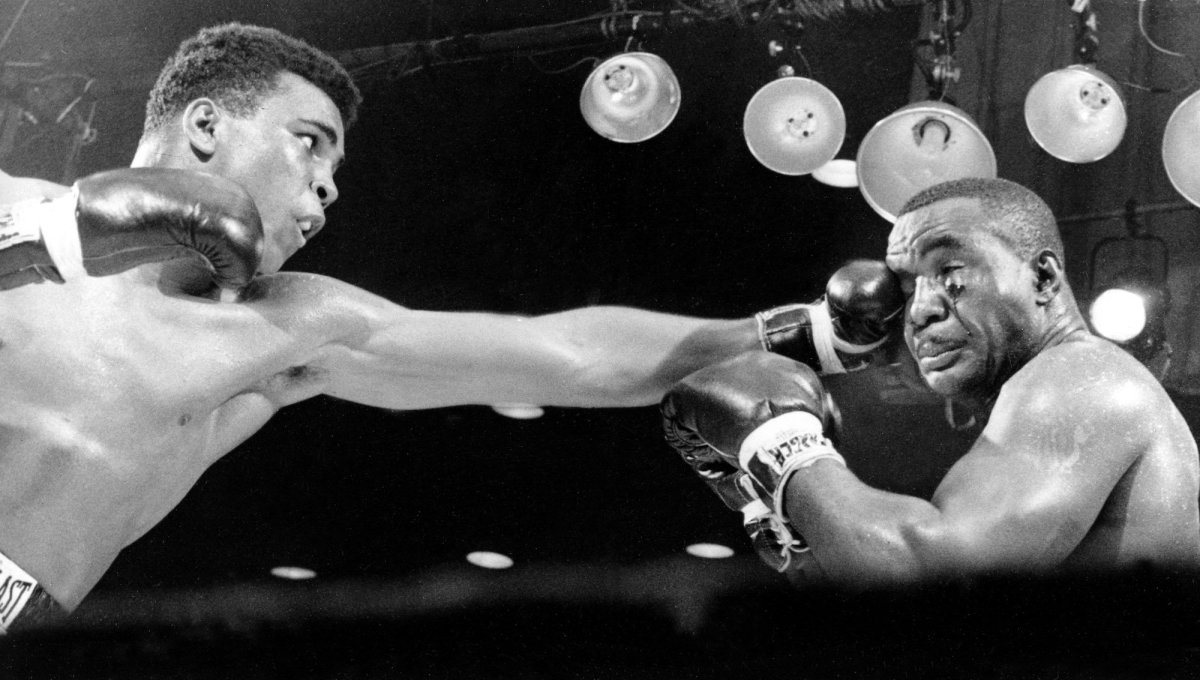A vintage black-and-white photograph captures a dramatic moment in a boxing match featuring a young Muhammad Ali. Positioned on the left, Ali is captured mid-action, delivering a powerful left punch directly to his opponent's right eye. The opponent, appearing battered with a noticeably swollen left eye, attempts and fails to adequately defend himself, his posture with bent elbows indicating he is struggling to withstand the blow. The scene is set in a boxing ring, with overhead lights illuminating the intense action, casting a stark contrast against the otherwise dark background, evoking the atmosphere of a 1960s boxing arena.